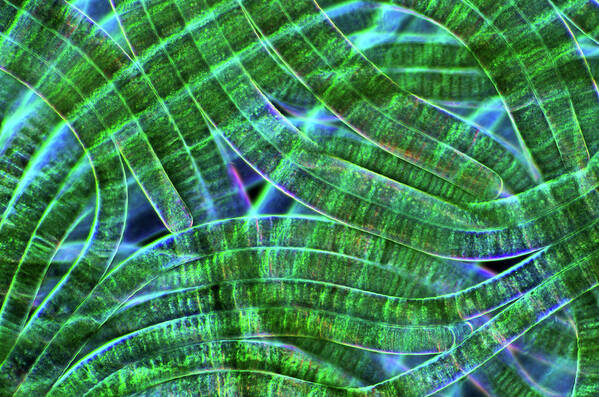This highly detailed, microscopic close-up image presents an intricate view, likely of a biological sample, possibly plant-based. The predominant color scheme showcases varying shades of green interwoven with delicate white outlines, resembling long, fibrous, worm-like structures or winding lines. These structures appear somewhat transparent, revealing turquoise and subtle purple hues illuminated beneath. The black background, though barely visible, accentuates the intricate network of these stacked green elements, creating a contrast that emphasizes the depth and complexity of the sample. The image, devoid of any text, appears to be taken with high magnification, such as from a microscope, illustrating what one might find in a biology textbook.